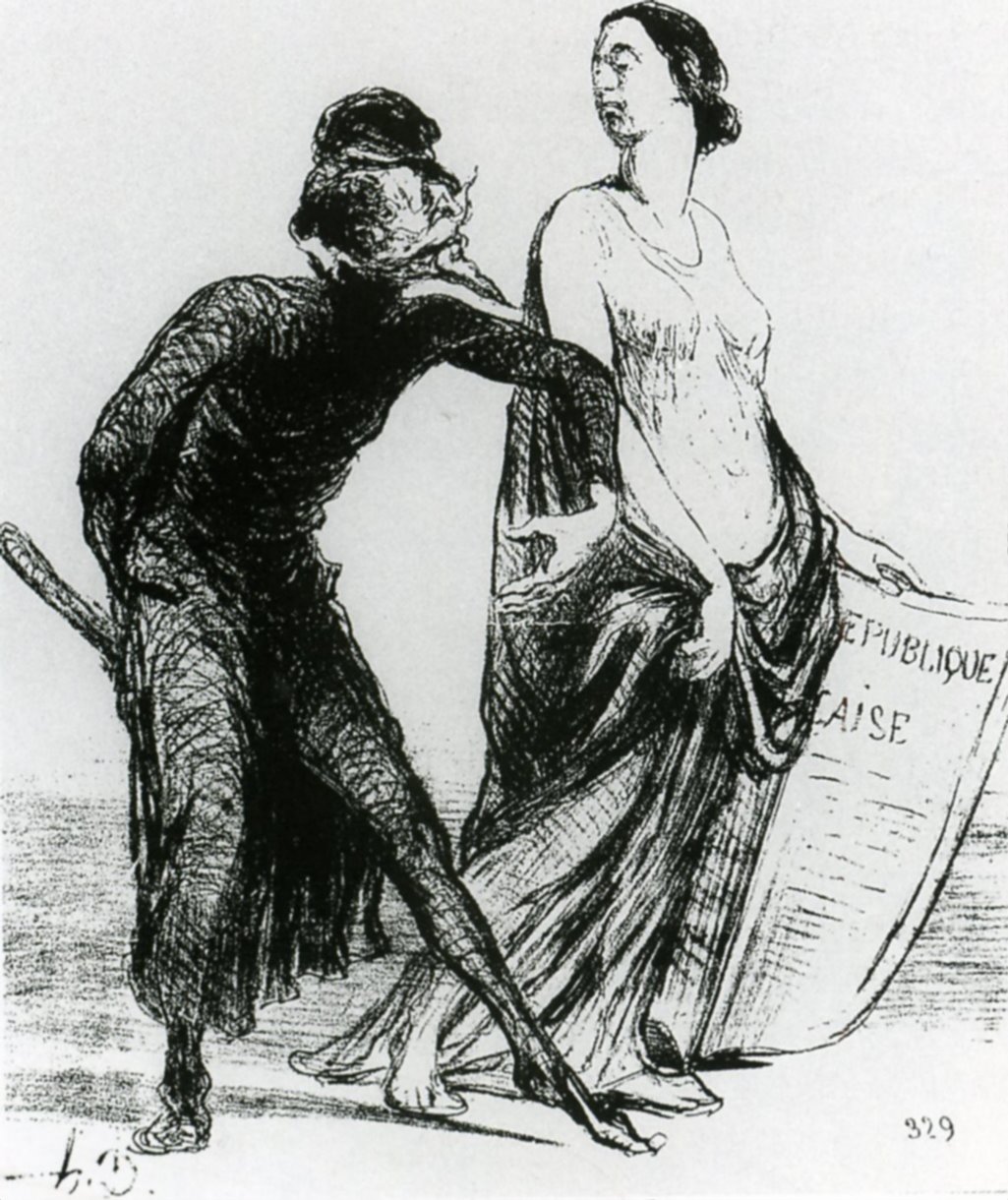This rectangular pencil sketch, approximately six inches tall and four inches wide, features two distinct figures set against a primarily light gray background, with heavier shading at the bottom suggesting a floor. The scene is set with a rather eerie atmosphere.

On the left, a man dressed entirely in black, with scratchy, pencil-marked attire, assumes a bent position extending his left leg forward and bending his right. His face, lined and aged, features a pronounced chin with facial hair, a pointy nose, and a dark cap atop his head. His expression is somewhat sinister, with sharp angles that add to his unsettling appearance. He reaches out with his left arm towards a woman, perhaps attempting to engage or seduce her.

The woman, positioned on the right, has her dark hair styled in a bun and appears to glance back at the man with a mix of disdain and apprehension. She is partially nude, outlined in light pencil marks, with a dark shawl draped over her, securing it at the front. In her left hand, she clutches a piece of paper or a sign that prominently reads "Republic," beneath which the letters "CAISE" or "LAISE" are partially visible, suggesting the text is cut off by her shawl. Her garments contrast sharply with the dark attire of the man, adding to the dramatic tension between the figures.

In the lower corners of the image, faint numbers and a nearly illegible signature appear, adding subtle details that enrich the sketch's complexity.